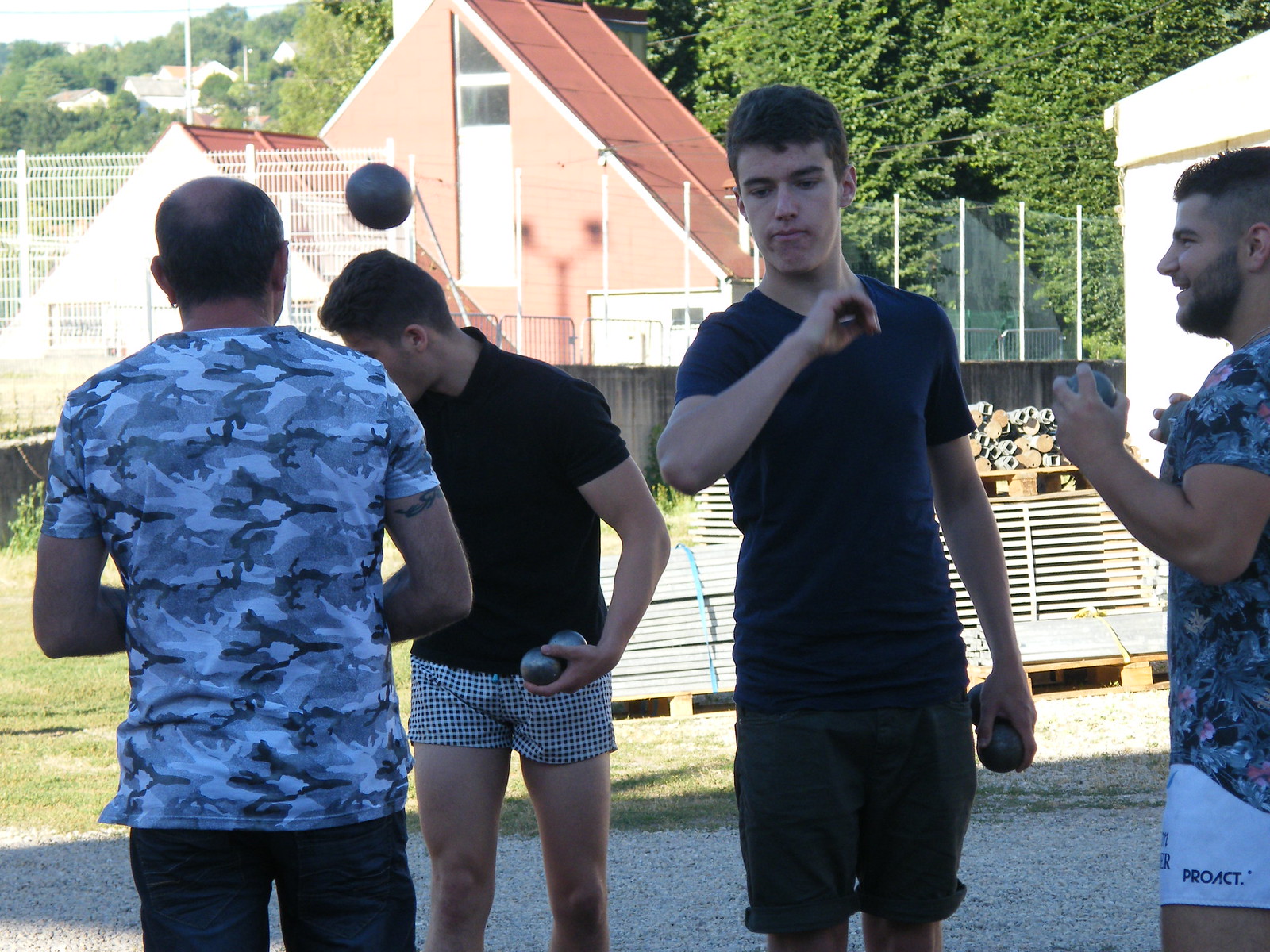On a bright, sunny day, a group of four men stands outdoors on a gravel surface, engaging in what appears to be a playful moment. The man closest to the left is facing away from the camera, obscuring his face and any other details about him. To his right, three men are visible, each holding several silver balls. The man on the farthest right has one shiny ball in each hand, exuding a calm stance. Next to him, a man holds two silver balls in one hand, showing a relaxed expression. The second man from the left, however, is the most animated, balancing two silver balls in one hand while tossing a third above his head, as if in mid-juggle. Their positions and expressions suggest a casual, light-hearted gathering, captured beautifully in the warm, natural sunlight.